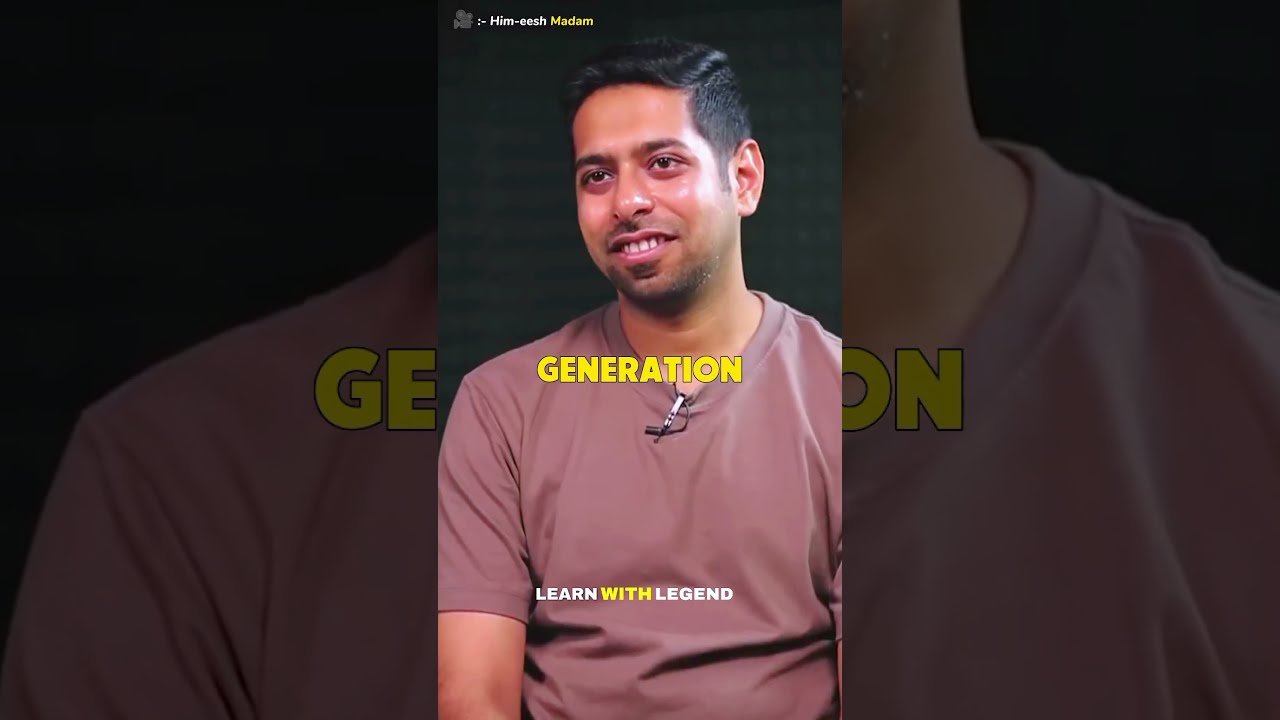This is a detailed photograph centered on a South Asian man with dark, neatly parted hair, styled short on the sides and slicked to the right. He has a warm smile revealing his top teeth and features a goatee. He wears a purplish-brown short-sleeved shirt with a microphone clipped to the neckline. The background is a green shade, slightly out of focus.

At the top of the image, small white text reads “Himish,” followed immediately by slightly smaller text that may read “Madam” in yellow font. A prominent yellow word, “Generation,” stretches across his neck and partial shoulder area. Below this, near the chest, the phrase “Learn with Legend” is displayed, with "Learn" and "Legend" in white font and "with" in yellow.

The left and right panels of the image are zoomed-in, slightly out-of-focus sections of the man’s shirt and neckline, creating a framed border effect. The left panel focuses on his right shoulder, showing the letters “GE” from the word "Generation," while the right panel captures part of his neckline and the shirt. Both panels emphasize the color and texture of his clothing, enhancing the central image's detail.